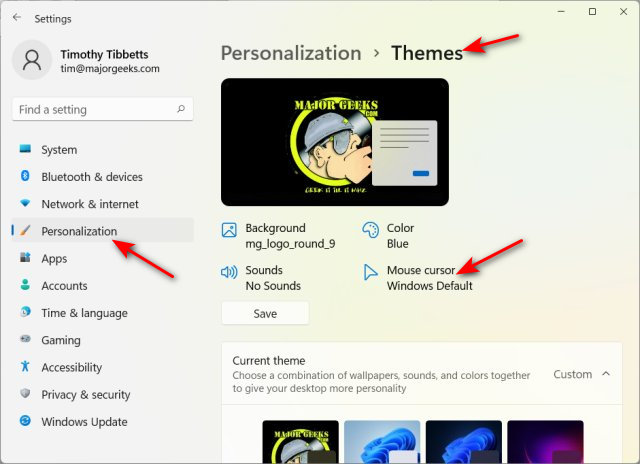The image is a screenshot taken from a computer screen, possibly from a web page or a settings program. In the top left corner, there is a header showing "Timothee Tibbetts" with the email address "Tim@majorgeeks.com". Below this, there is a profile icon that is a generic human figure. The left sidebar lists various settings options including System, Bluetooth & devices, Network & Internet, Personalization, Apps, Accounts, Time & Language, Gaming, Accessibility, Privacy, Security, and Windows Update. The Personalization section is selected. 

In the main part of the screen, the title "Personalization" is displayed prominently with a subheading "Themes". A red arrow points to the word "Themes". Below this is a black rectangle resembling a business card, featuring a cartoon logo with the text "MajorGeeks.com". The rectangle lists options such as background, color, sound, and mouse cursor, with another red arrow pointing to "Mouse Cursor: Windows Default". The image seems to be instructing on the personalization settings of a computer, detailing different customization options available to the user.